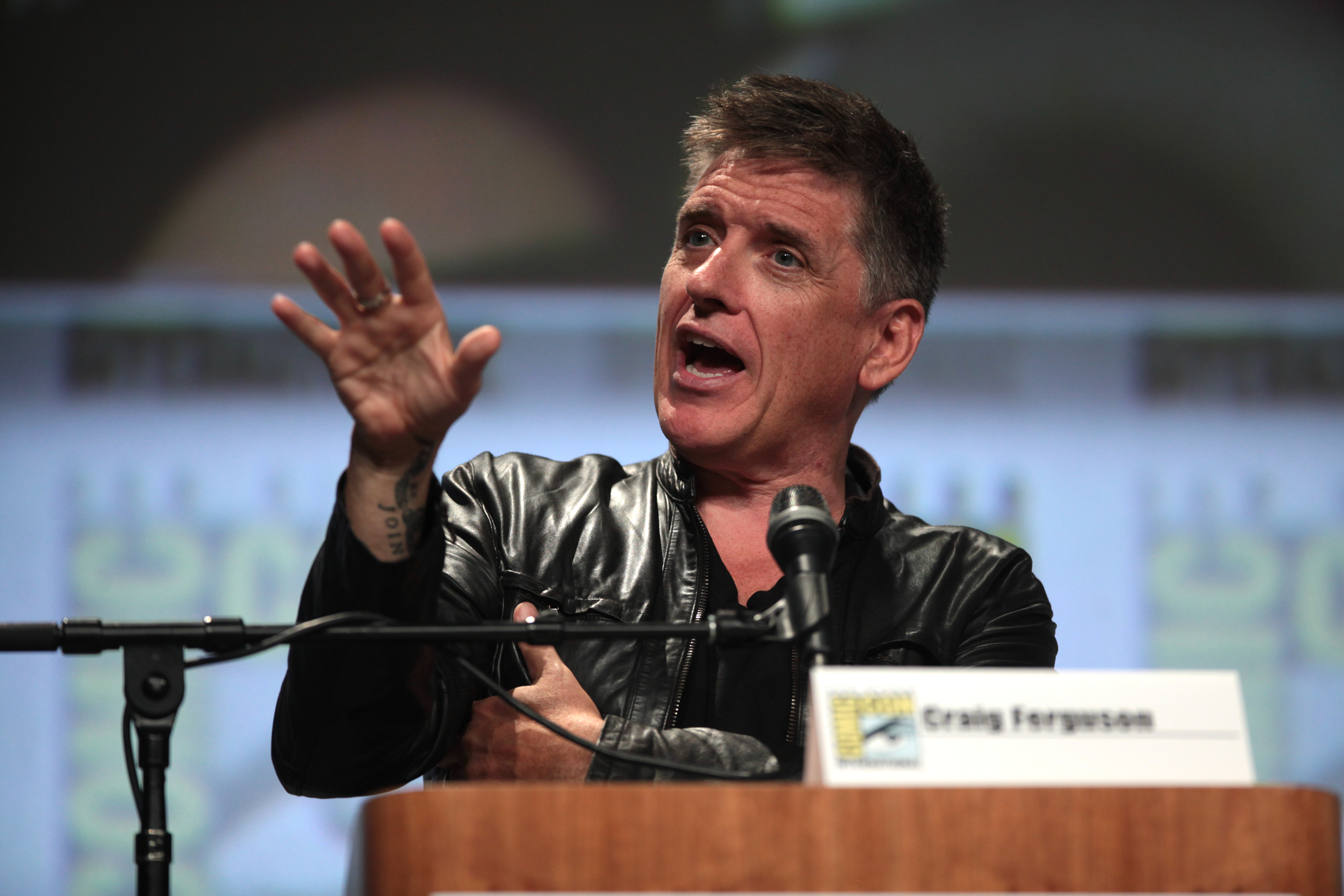The image depicts an indoor event, possibly a speech or engagement, with a man prominently featured at the center. The background is out of focus, showing a blend of colors—gray, yellow, blue, and black—with what looks like some blurry text and partial banners. The man, identified by the name tag on the wooden podium as Craig Ferguson, wears a black leather jacket. He is speaking into a microphone positioned at neck level, with his right hand raised in a gesturing manner and his fingers splayed apart, displaying a ring on his middle finger and revealing a tattoo. His left hand is wrapped across his chest, tucked somewhat under his raised right hand. Craig's mouth is open as he addresses the audience, and he has short, trimmed brown hair and dark brown eyes. The blurred yet colorful backdrop contrasts with the sharp focus on Craig at the podium, highlighting his expressive gesture and engagement with the audience.